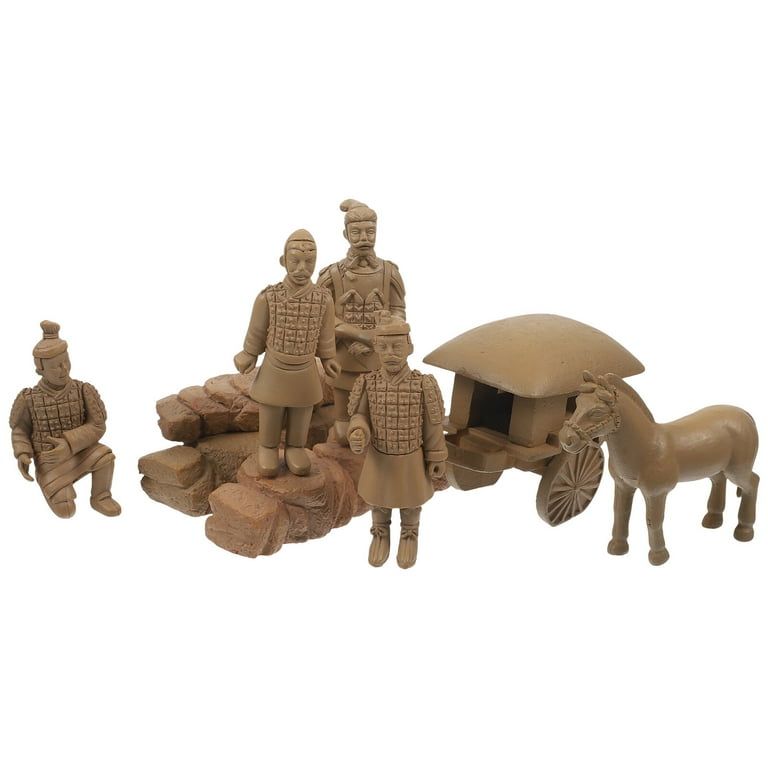The image features a series of detailed figurines likely representing an ancient Asian tableau, possibly from China or Indonesia. The scene includes four human figures, a horse, and a covered wagon. The figurines are crafted from a smooth, shiny material resembling plastic or carved stone, all uniformly colored in a brownish-gray hue, while their base features reddish-brown rocks. 

The humans, appearing distinctly old-time, are adorned in patterned attire, with most wearing square-patterned shirts paired with skirt-like tunics, long pants, and boots. One figure stands out with V-patterned squares on his shirt, shoulder armor, and a unique headpiece that resembles either a Santa cap or a topknot. He's positioned at the back. 

To their side, there's a horse standing next to a wagon, which sports a domed cover and spoked wheels. The thoughtful arrangement includes a kneeling figure on the left, and two men standing on rocks to the right. The man in front of the rocks is posed with his arm bent forward, as if greeting someone. The wagon faces the men, while the horse or donkey underneath it faces left, its tail down. The backdrop of the image is plain white, ensuring all attention remains focused on these intricate figurines.